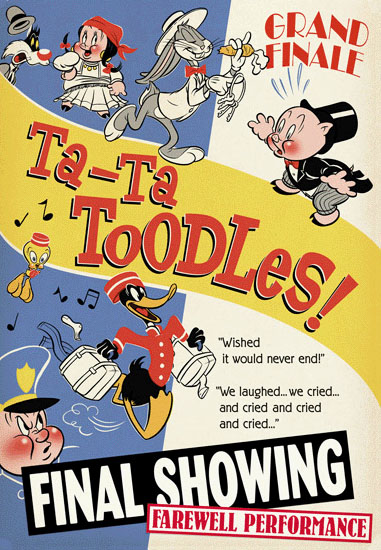This old-time poster from the Warner Brothers collection advertises a grand finale show, featuring a blend of beloved cartoon characters from the Looney Tunes universe. The left side of the poster has a purplish-bluish background that becomes narrower towards the bottom, while the right side features a white background that widens at the bottom. Dominating the upper left corner is Sylvester the Cat, with a gray hat flying off his head. Below Sylvester is a porcupine-like character wearing a white dress and an orange scarf.

Central to the composition is Bugs Bunny, positioned slightly off-center. Bugs is depicted in a white hat and white suit with a red bow tie, holding a ring of keys in one hand and a carrot in the other, walking towards the right side of the page. Directly ahead of Bugs is Porky Pig, who assumes the role of a ringleader, adorned in a tall black hat, black suit with tails, and gray pants. Above Porky Pig's head in large red letters against a white background are the words "GRAND FINALE."

A prominent yellow band runs horizontally across the center, featuring the red-lettered message "Ta-Ta Toodles!" alongside two musical notes. Below this yellow band, additional musical notes are seen, coupled with the phrase "WISHED IT WOULD NEVER END, WE LAUGHED, WE CRIED, AND CRIED, AND CRIED, AND CRIED." Further below, in a black box with white lettering, it says "FINAL SHOWING," and beneath it in a white box with a red border and red letters, it states "FAREWELL PERFORMANCE."

To the right of the poster and positioned on top of the yellow band is another figure of Porky Pig, dressed in a top hat and tails, reinforcing his ringleader persona. Tweety Bird is below and left of the yellow band, dressed as an usher with a red pillbox hat, and nearby is Daffy Duck in a bellboy uniform with a matching red hat, carrying two white suitcases. In the lower left corner of the blue section, a stern-looking policeman with red rosy cheeks, a blue hat with a gold shield and band, and a black visor completes the vivid tapestry of characters. With its rich array of detailed illustrations and vibrant textual elements, the poster captures the nostalgic charm and dynamic excitement of a farewell performance for these iconic characters.